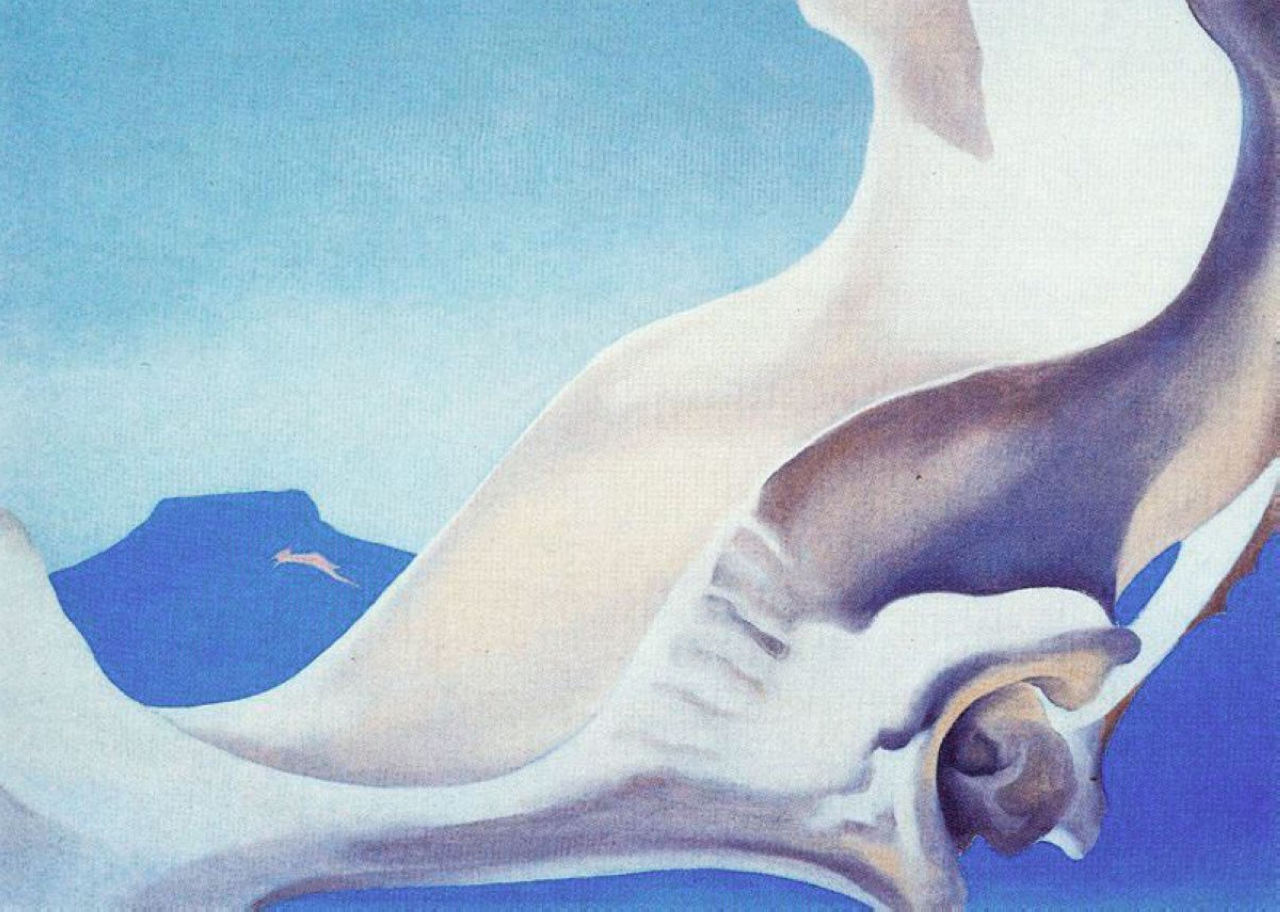This intriguing painting, open to interpretation, showcases a modern, flowing style reminiscent of bright pastels. Dominated by shades of blue, white, and gray, the most prominent feature is a large, central object that could resemble a bird's wing or a shell's structure. This object, seemingly smooth with curved designs and wavy lines, spans diagonally from the lower left to the upper right, filling the canvas. In the background, a serene blue mountain fades into a light blue sky with soft, cloud-like patterns, blending gently into the mountainous horizon. Below what may be the head of a bird or another mysterious creature, the canvas transitions into a tranquil blue, evoking a sense of both air and sea. The painting's soothing colors and ambiguous forms compel viewers to contemplate its meaning, making it a captivating and serene piece of art.